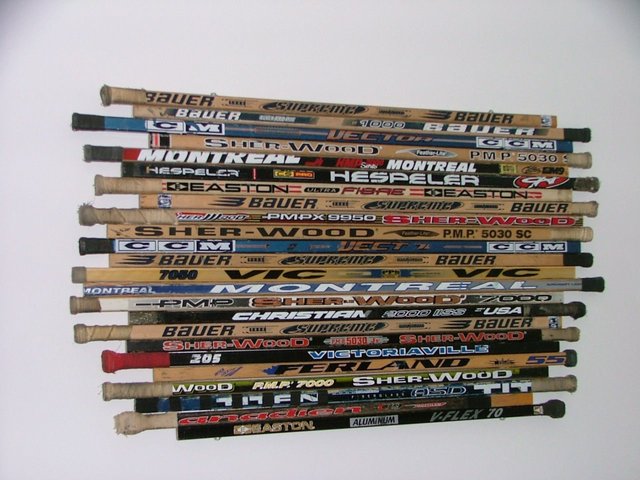The image showcases an assortment of hockey sticks mounted on a gray wall, each positioned flatly on top of one another. The collection features an array of sticks, predominantly wooden with some colored ones interspersed, each bearing distinct brand names and lettering. Prominently, the brands "Bauer," "Sherwood," "Christian," "Montreal," and "Easton" can be seen among many others. The sticks appear worn, with some sporting tattered athletic tape around their handles, indicating frequent use. The scene offers a fascinating look at the variety of hockey sticks, boasting both wooden and colored finishes, set against a light gray backdrop.